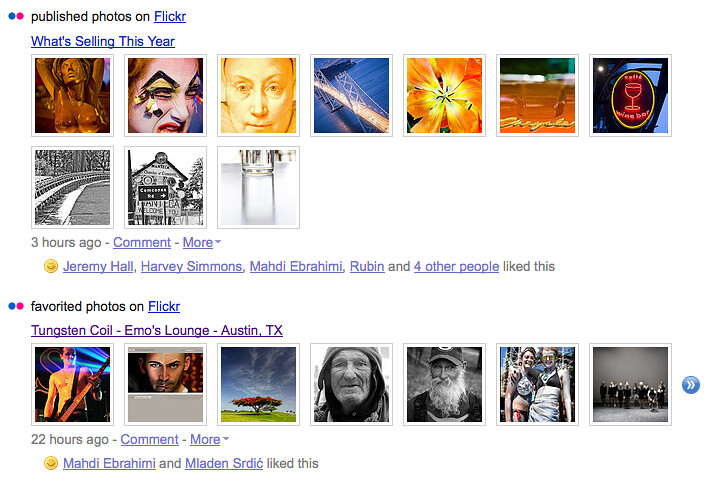This detailed screenshot from Flickr showcases a collection of images posted by various users. At the top of the screenshot, the text reads "Publish photos on Flickr," followed by a clickable link titled "What's selling this year?" Below this, there are two rows of images: the first row consisting of seven small icons or thumbnails of diverse photos, including portraits, flowers, railroad tracks, a house, and a bronze statue of a topless woman, among others. The second row contains three smaller photos.

Directly underneath these rows, there is information about user interactions: "three hours," followed by "comment more," and the names "Jeremy Hall, Harvey Simmons, Monty Ibrahimi, Ruben, and four other people like this."

Subsequently, another section begins with the title "Favorite photos on Flickr" in purple. Below this, it specifies "Tungsten Coil, Emo's Lounge, Austin, Texas." This section also contains two rows of seven images each, featuring a variety of subjects, such as a stage performer, a person, a tree, multiple portraits, and two individuals with bras over their clothes hugging each other. The final line mentions that the post is "22 hours" old, with users "Monty Ibrahimi and Madden Shreddick" liking it.